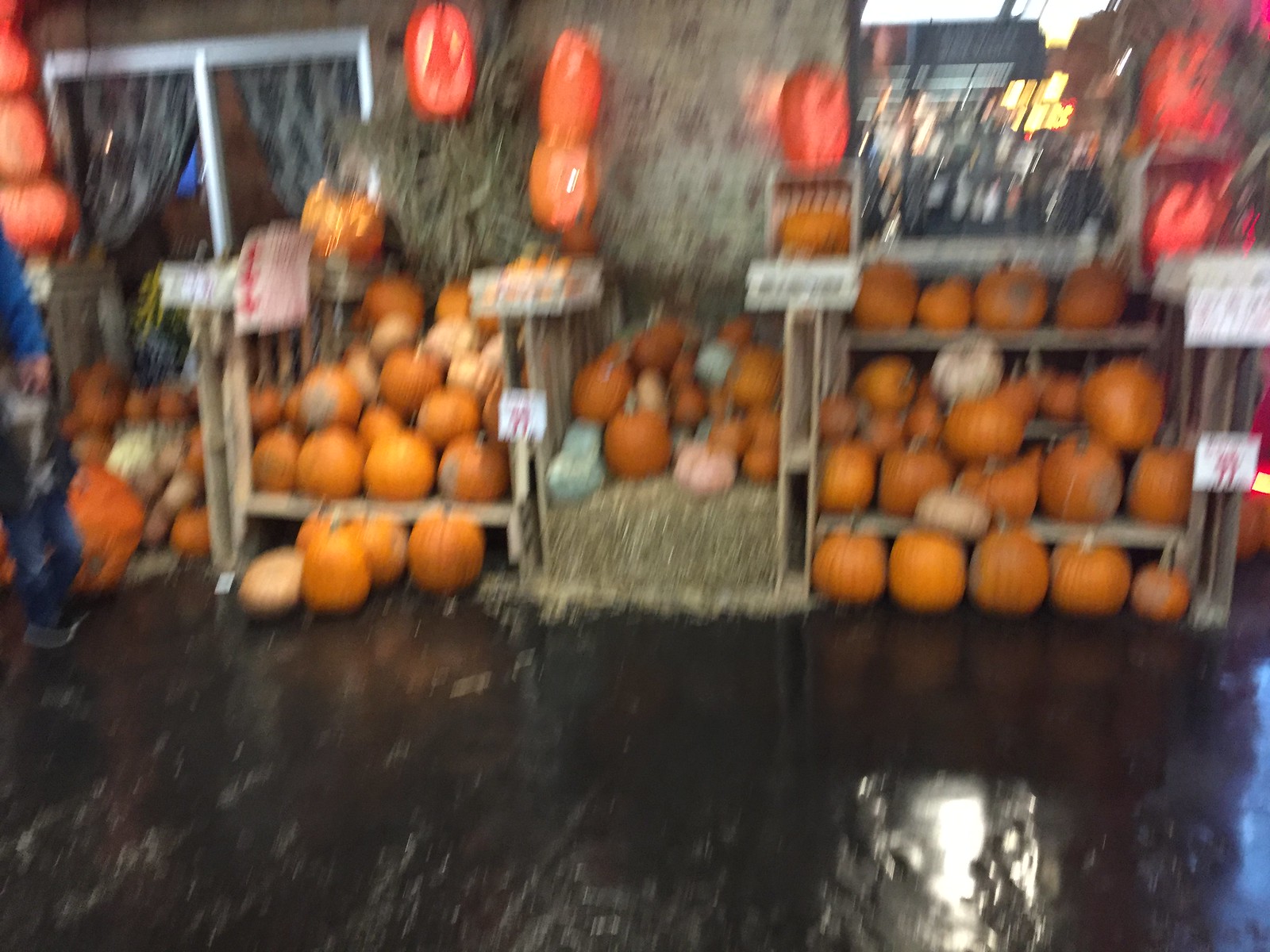This photograph, though blurry, captures a bustling market scene replete with festive autumn decor. At the bottom of the frame, a glossy black floor appears wet, reflecting bright lights and adding a dramatic shimmer to the scene. Above the floor, a rustic brown brick wall serves as a backdrop for an array of pumpkin displays. In the center, a beige hay bale acts as a pedestal for a neatly piled stack of pumpkins. To either side of this centerpiece, wooden stands overflow with large, vibrant orange pumpkins, contributing to the abundant harvest theme.

Suspended from the top of the frame are round, illuminated jack-o'-lantern lamps, casting a warm glow over the displays. On the left, a silver-rimmed black glass door or window stands behind one of the pumpkin arrangements, while on the right, another window reflects a brightly lit cityscape, adding an intriguing urban contrast to the rustic market setting. Despite the blurriness, the photograph conveys a lively, festive atmosphere in celebration of the autumn season.